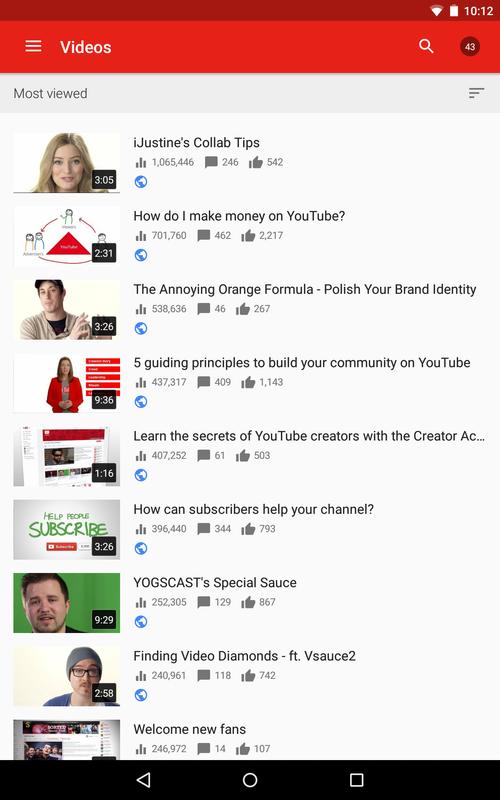A cell phone screenshot displaying a video browsing interface. The top section of the screen is highlighted in red and burgundy hues, indicating active menu categories. The timestamp reads 10:12, and the battery icon shows a nearly full charge.

The header includes three horizontal lines near the word "Videos" and a clickable search magnifying glass icon. Below the header, the section labeled "Most Viewed" showcases a list of nine videos, though the ninth is partially cut off due to screen size constraints.

Each video entry features a thumbnail image on the left side, providing a glimpse of the video's content. In the lower right corner of each thumbnail, a black box with white text indicates the video's duration. Central to each entry is the video's title, flanked by various interactive icons such as thumbs up and comment options, allowing for user engagement.